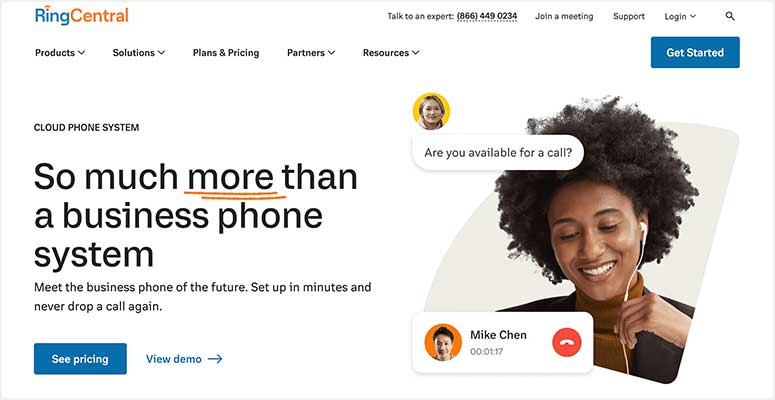The image features a clean, white background with a central focus on the branding elements of "Ring Central"—where "Ring" is highlighted in blue and "Central" in orange. Prominent call-to-action buttons are displayed, including "Talk to an Expert: 866-449-0234," "Join a Meeting," "Support," "Log In," and a magnifying glass icon. A blue button labeled "Get Started" in white text is also visible.

The image emphasizes a range of product offerings and services: "Product Solutions," "Plans and Pricing," "Partners," and "Resources," alongside features like "Cloud Phone System" and "So much more than a business phone system." A headline in bold promises, "Meet the Business Phone of the Future," with subtext highlighting quick setup and reliable call quality.

A notable blue rectangle button that reads "See Pricing" in white is accompanied by another that says "View Demo." The text "Mike Chin, 00-01-17" appears next to a red circle icon indicating an active call, showing a small picture of a man. 

In the foreground, a yellow circle encloses an image of a woman asking, "Are you available to call?". The woman is dressed in a black suit with a gold turtleneck, wearing an earphone and smiling while looking at a device, possibly a phone. Her smile reveals her teeth, adding a friendly and professional touch to the image.